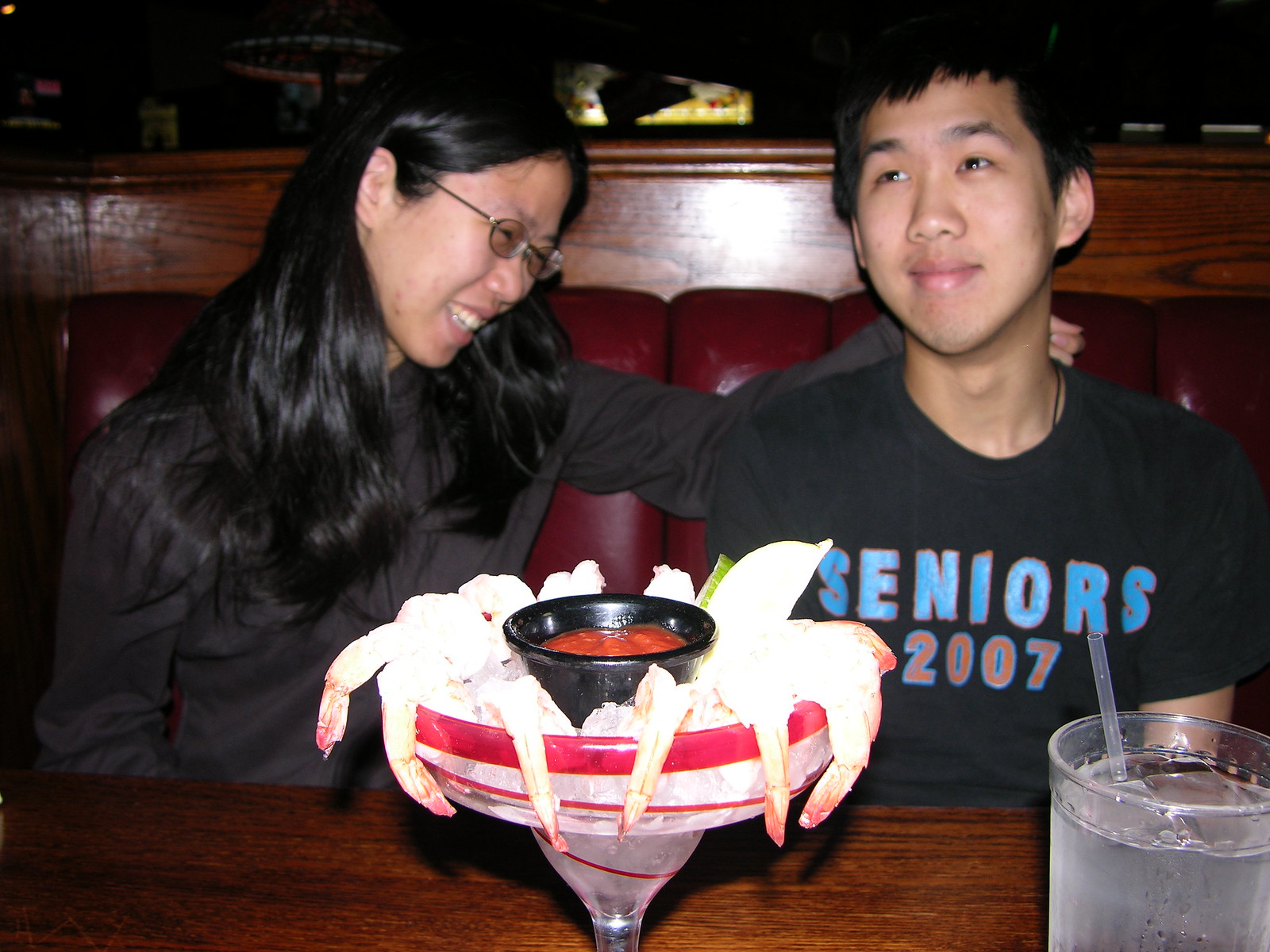This is a detailed color photograph of a man and a woman sitting together in a restaurant booth with red leather upholstery and a wooden top edge. They are seated at a dark brown wooden table. The woman, who appears to be Chinese, has long black hair and is wearing a black sweater. She also has glasses and is smiling with her left arm draped over the shoulders of the man next to her. The man, also appearing to be Chinese, is wearing a black t-shirt with the words "Seniors 2007" printed in blue and red font. He is looking up to his right and smiling. In front of them on the table is a shrimp cocktail in a large clear glass with red stripes, garnished with big pieces of shrimp hanging off the side, and a small black container of red sauce in the center. In the bottom right corner of the image, there is a glass of iced water with a clear straw. The background appears mostly dark, contrasting with the bright red and wooden elements of the booth and table.